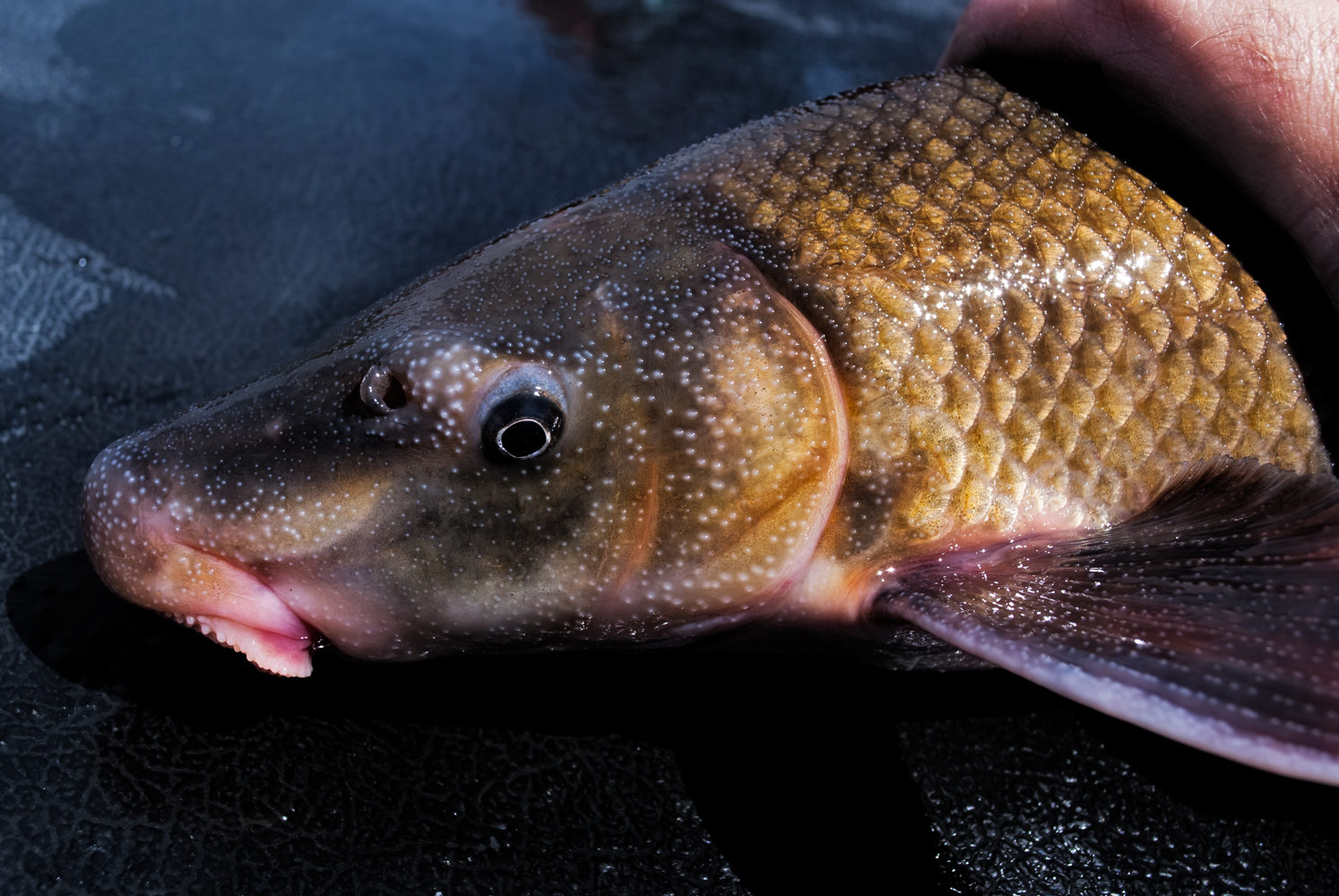The image depicts a close-up of a fish, seemingly caught and no longer alive, lying on a dark, possibly black leather surface, likely in a boat. The fish is primarily golden-green, with dark yellow scales transitioning into a dark green and black head, adorned with small blue dots. The eye on the left side of the image is black with a white ring around it. The fish's lips appear pink, and there is a light purple edge on a visible purple fin. A hand is holding the fish down by its side fins, making it clear that someone has caught it but it is unclear whether it will be released back into the water.